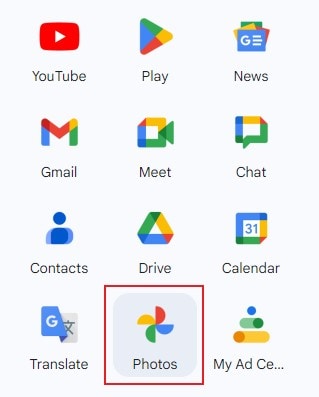This image showcases a cropped screenshot of a smartphone screen, specifically capturing a portion of the app grid. The visible section of the screen is not the entire display and measures three icons in width, contrary to the more typical four-wide arrangement found on most smartphones. The background is a clean white, and no status bar details like time or battery life are visible at the top. The icons are displayed with their respective names underneath them, each featuring its recognizable symbol.

In the first row of icons:
- YouTube

In the second row:
- Play Store (labeled as "Play")
- Google News (labeled as "News")

In the third row:
- Gmail
- Google Meet (labeled as "Meet")
- Google Chat (labeled as "Chat")

In the fourth row:
- Google Contacts (labeled as "Contacts")
- Google Drive (labeled as "Drive")
- Google Calendar (labeled as "Calendar")

In the fifth row:
- Google Translate (labeled as "Translate")
- Google Photos (labeled as "Photos")
- An unfamiliar app labeled "My Ad"

The Google Photos icon is highlighted, indicating it has been selected. The cohesive design and labels suggest a focus on Google apps, providing a glance at some of the essential tools and services from the tech giant.